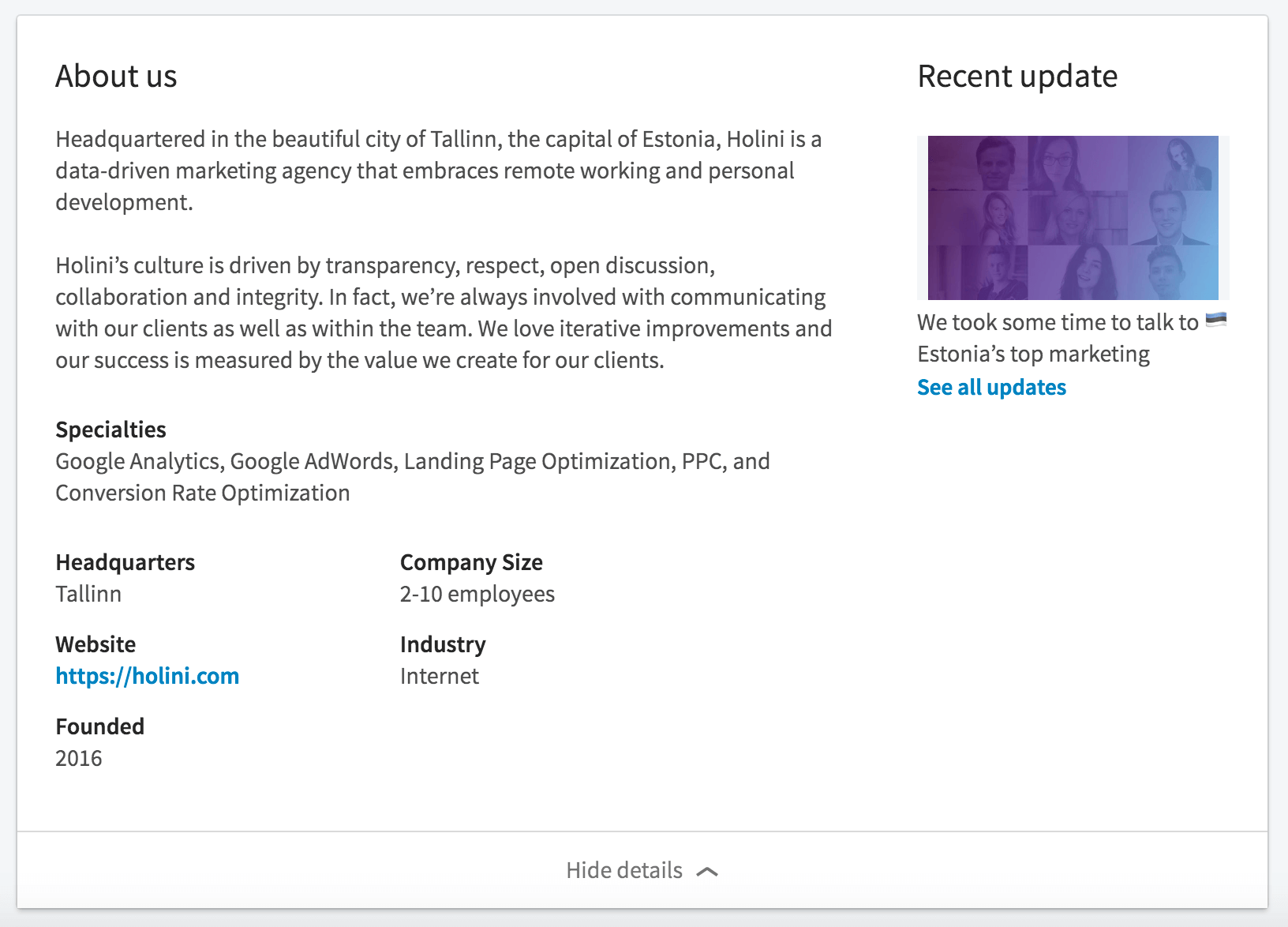This image is a screenshot from a webpage with a white background. In the upper left-hand corner, the text "About Us" is written in gray font. Below this, it states that the company, Holini (H-O-L-I-N-I), is headquartered in the beautiful city of Tallinn, the capital of Estonia. Holini is described as a data-driven marketing agency that embraces remote work and personal development. 

The description continues beneath this section. Under the headline "Specialties," it lists Google Analytics, Google AdWords, landing page optimization, PPC (Pay-Per-Click), and conversion rate optimization. Additional details include that the company's headquarters is in Tallinn and it has a size of 2 to 10 employees. The website provided is H-O-L-I-N-I.com, and it was founded in 2006.

In the upper right-hand corner, under the headline "Recent Update," a purple square is visible, which contains an overlay of stock photos featuring headshots of people. Below this image, it states, "We took some time to talk to Estonia's top marketing...," signaling an incomplete message. Further below, there is a blue link with the text "See all updates."